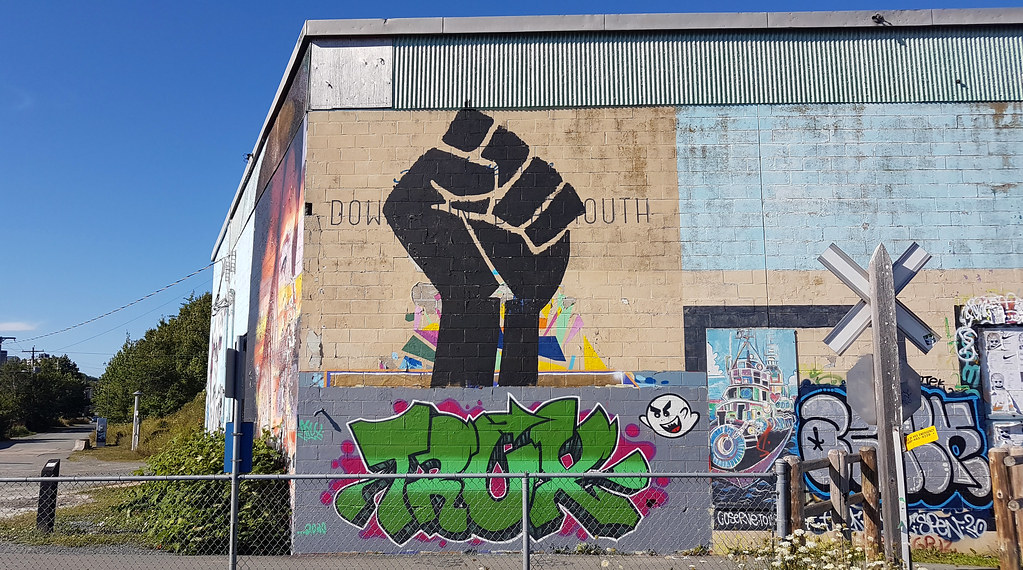The image showcases a tan cinder block building adorned with various types of graffiti, set against a brilliant blue sky occupying the upper left corner and stretching horizontally across the scene. The building features a distinct black fist centrally painted on the wall, partially obscuring letters that appear as "BOW" at the beginning and are cut off towards the end. To the right of this, a blue rectangle adds a splash of color. The lower portion of the wall displays vibrant, multi-colored graffiti with shades of green, purple, blue, yellow, and lighter green forming abstract shapes and designs. Below this artwork, the word "TRUX" is spray-painted in green, capital letters, reminiscent of a graffiti tag. In front of the building, a gray railroad crossing sign stands, with its stem planted firmly into the ground amidst an untidy landscape, peppered with scattered debris, grass, and patches of trees, further suggesting a neglected, rundown area.